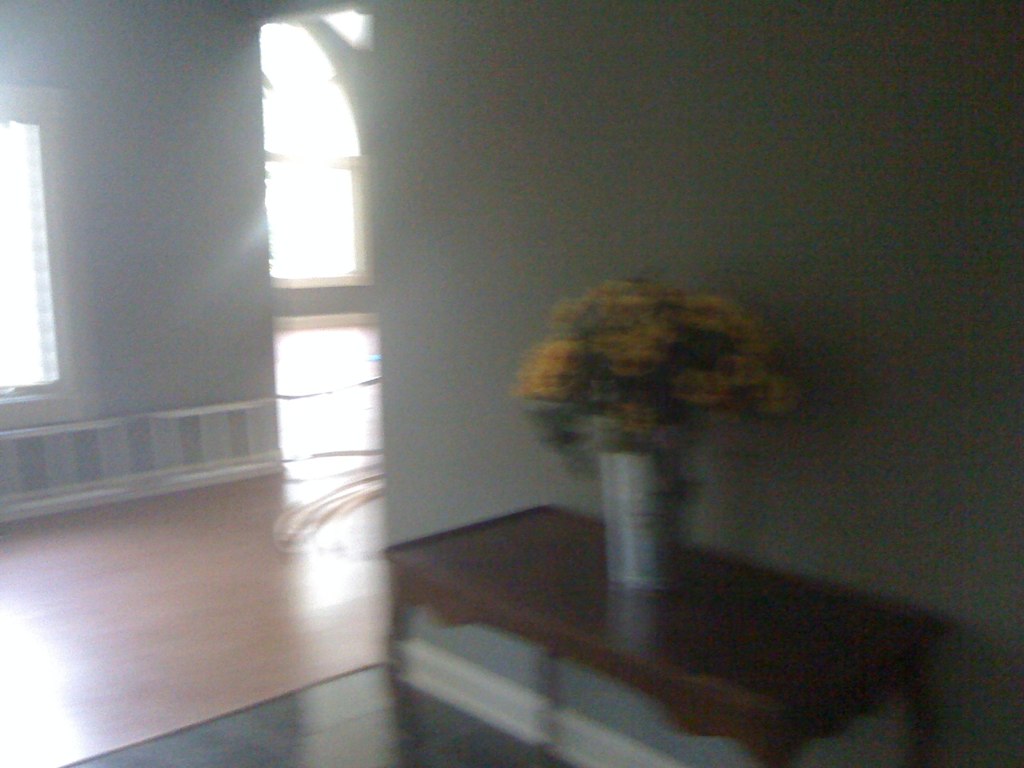In this photograph of an indoor setting, the room appears dimly lit despite the presence of some bright lights and illuminated windows in the background. The overall ambiance is somewhat dark, accentuated by noticeable motion blur and considerable digital noise, giving the impression that the room's lighting was insufficient when the picture was taken. The walls of the room are painted a muted gray. In the bottom right-hand corner, a brown wooden table stands against the wall. Atop this table rests a metallic vase or canister, which holds a vibrant bouquet of yellow flowers with lush green stems, adding a touch of color and life to the subdued surroundings.